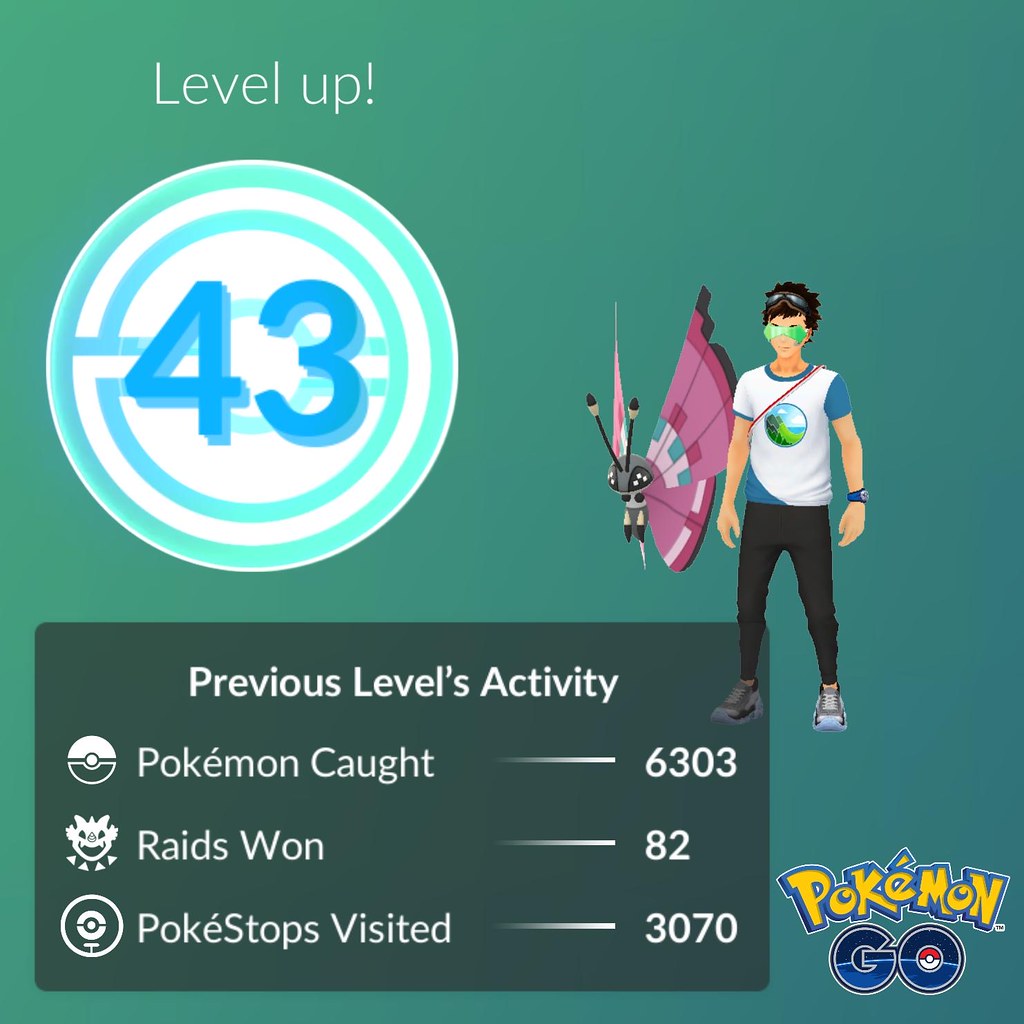The image is a detailed screenshot from the mobile game Pokémon Go, capturing the moment when a player’s Pokémon levels up. The background is a dark teal color. In the upper left corner, the words "Level Up!" are prominently displayed in white. Below this, a large white circle with green rings frames the level-up number, which is 43, depicted in bold blue. To the right of the level number, there is a digital illustration showcasing the player's avatar: a man in black pants, a white t-shirt, and sunglasses. He stands next to a purple Pokémon. 

Along the bottom of the image is a large black rectangle displaying a summary of the player's statistics in white text. It highlights the "Previous Levels Activity," showing that the player has caught 6,303 Pokémon, won 82 raids, and visited 3,070 Pokéstops. In the lower right corner, the Pokémon Go logo is visible, confirming the game's branding.